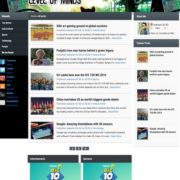A vertically oriented image, approximately 20% taller than it is wide, presents a blurry, zoomed-out excerpt of a web page. The image is somewhat cropped on the sides, giving an impression of being very small. At the top, a faint banner serves as the backdrop, possibly featuring the head of a black cat centrally. Surrounding the cat is a blend of green and yellow hues. Text at the top left reads "level of," but the final word is unreadable, consisting of approximately five to six black-colored characters.

The main section below showcases a gray background. On the left side, a navigation menu displays about seven to eight lines of white text, too diminutive to decipher. This menu is punctuated by six icons aligned vertically, each accompanied by gray text to the right. The central area features five square images aligned vertically on the left. Adjacent to them on the right is a bolded heading, followed by a smaller, unreadable body of text.